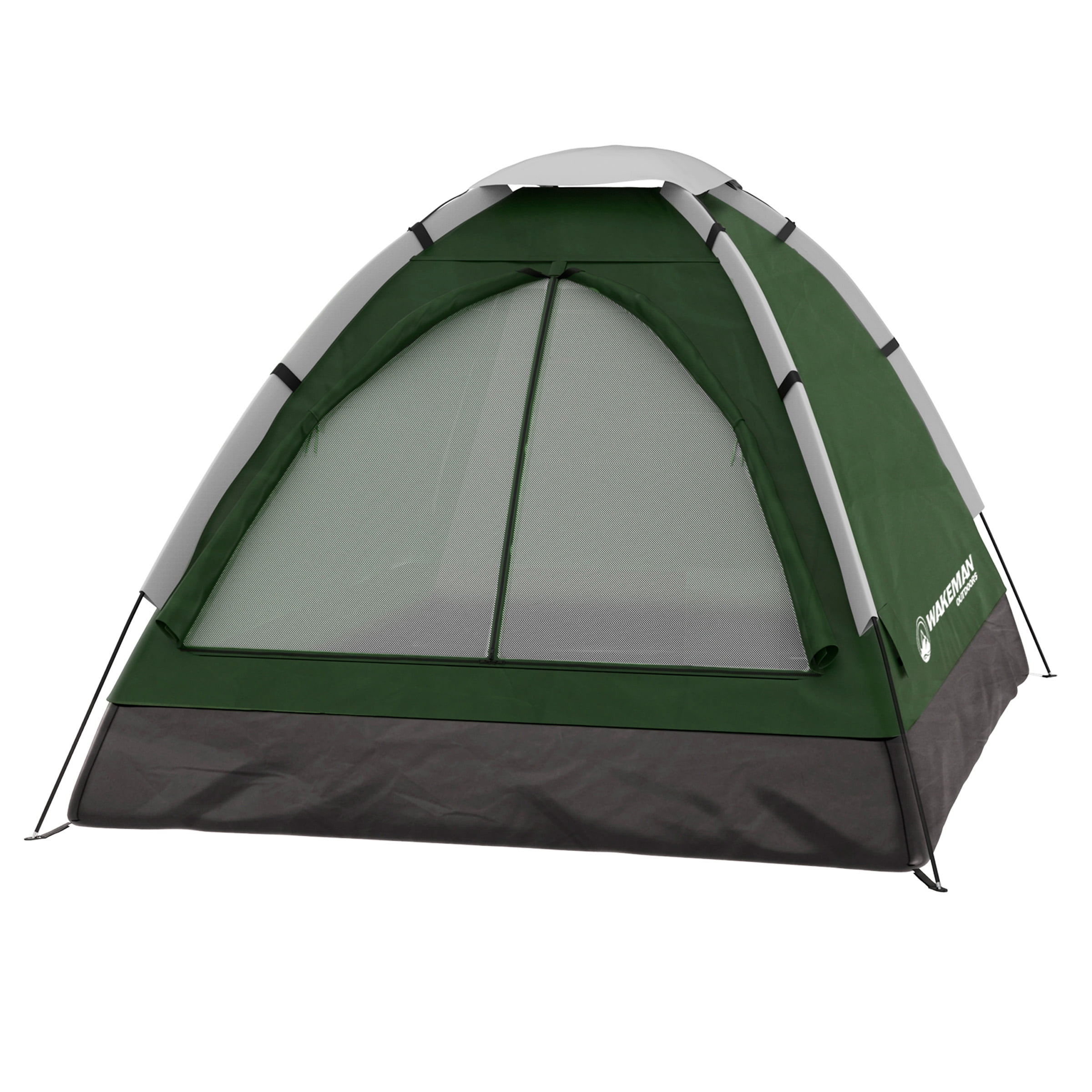This promotional image features a modern dome-shaped camping tent set against a completely white background. The tent showcases a two-tone color scheme: the top 80% is green, while the base is a dark brown or black nylon material. Four black metal rods arch around and connect the tent, secured by canvas loops to maintain its structure. These rods are partially covered by white protective sleeves. The tent includes a top hood designed to keep rain off the dome. The front has a zippered door, which is gray with a brown zipper, and appears semi-transparent, hinting at the interior. On the right-hand side, the brand name "Wakeman" is visibly printed in white, accompanied by a logo.